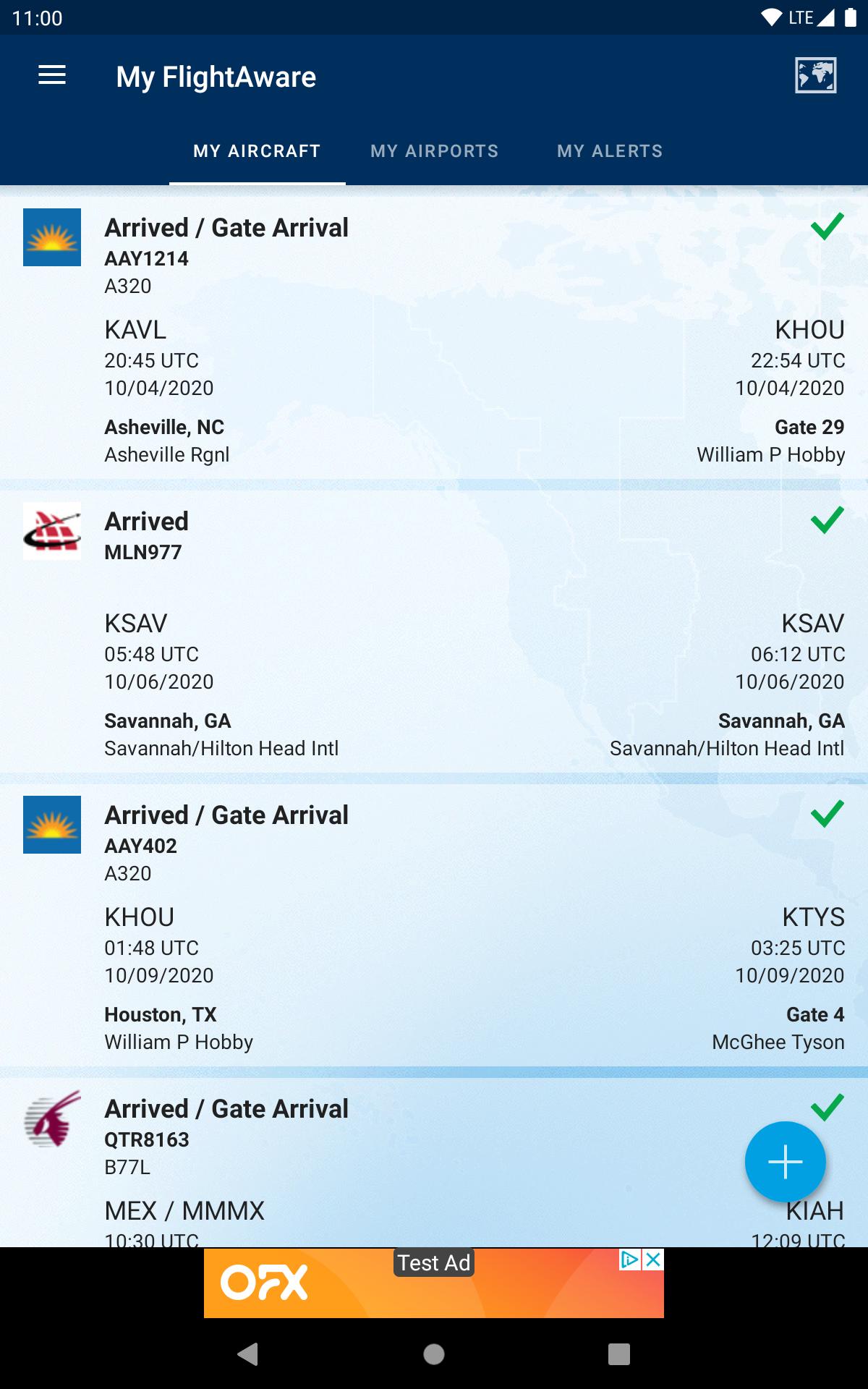Screenshot captured on an Android phone at 11:00 AM. The status bar shows a Wi-Fi connection, LTE connectivity with full signal bars, and a fully charged battery. The image displays a flight tracking application, specifically the "My Flight Aware" section. There are three clickable headers: "My Aircraft," "My Airports," and "My Alerts," with "My Aircraft" currently selected.

Within the "My Aircraft" section, there are four visible entries:

1. **Arrived / Gate Arrival**:
   - **Flight**: AAY-1214 (A320)
   - **Route**: Asheville Regional Airport (KAVL) to William P. Hobby Airport (KHOU)
   - **Date & Time**: October 4, 2020, arriving at 20:45 UTC in Asheville and landing at 22:54 UTC at KHOU
   - **Gates**: Gate 29 at Asheville
  
2. **Arrived**:
   - **Flight**: MLN-977
   - **Route**: Savannah/Hilton Head International Airport (KSAV) to KSAV
   - **Date & Time**: October 6, 2020, from 05:48 UTC to 06:12 UTC
   - **Location**: Savannah, Georgia
  
3. **Arrived / Gate Arrival**:
   - **Flight**: AAY-402 (A320)
   - **Route**: William P. Hobby Airport (KHOU) to McGhee Tyson Airport (KTYS)
   - **Date & Time**: October 9, 2020, from 01:48 UTC to 03:25 UTC
   - **Gates**: Gate 4 at McGhee Tyson Airport
   - **Location**: Houston, Texas to Knoxville, Tennessee

4. **Arrived / Gate Arrival**:
   - **Flight**: QTR-8163 (B77L)
   - **Route**: Monterrey International Airport (MMX) to George Bush Intercontinental Airport (KIAH)
   - **Date & Time**: 10:30 UTC to 12:09 UTC